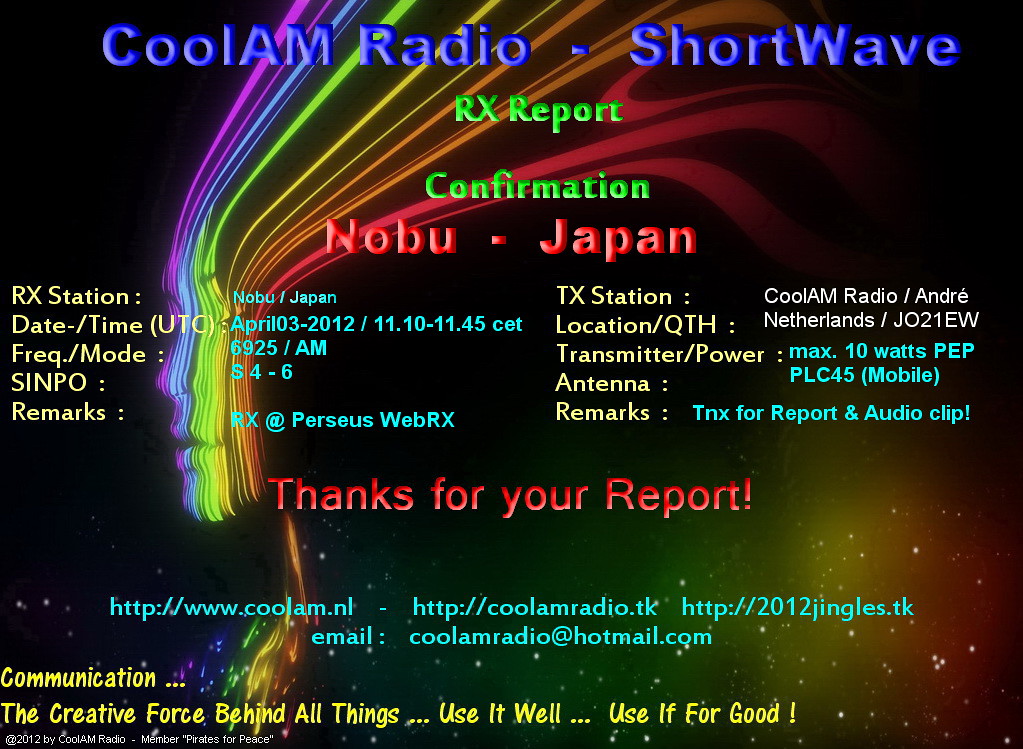The advertisement features a striking, surreal artistic composition with a black background. Dominating the imagery is the left profile of a woman's face created from vibrant, undulating ribbons of color—red, orange, yellow, green, blue, and purple—that stretch from the top to the middle bottom of the image, extending into her neck. These colorful lines form a captivating, rainbow-like portrayal of the face set against a backdrop that turns into a haze of sparkly rainbow hues toward the bottom.

At the top of the advertisement, text in bold, multi-colored fonts reads "Cool AM Radio / Shortwave RX Report Confirmation Nobu Japan." Beneath this headline, additional details are provided in similarly vibrant fonts: "Date: April 3rd, 2012, 11:10 to 11:45 CET," "Frequency Mode: 6925 AM," "Remarks: RX at Perseus Web RX," and "Thanks for your report: http://www.coolam.nl." Further information about the transmission includes the "RX Station: Nobu Japan" and "TX Station: Cool AM Radio Andre," with location details stating "Netherlands J021" and "Transmitter Power: Max 10 watts PEP Mobile."

A motivational message at the bottom, highlighted in yellow font, reads: "Communication: The Creative Force Behind All Things. Use it well, use it for good."